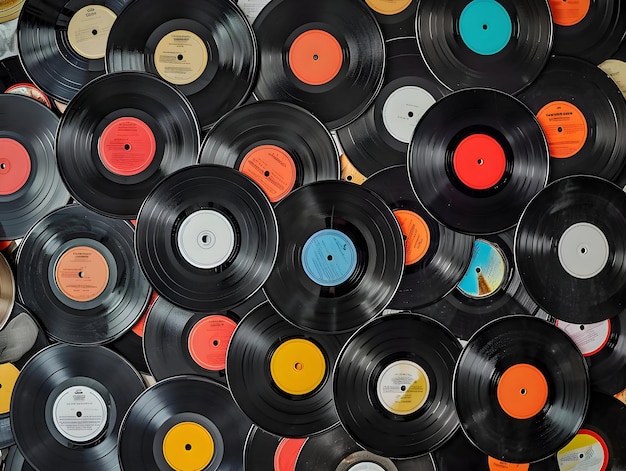This vibrant image is filled with an array of stacked vintage vinyl records, each with a colorful label at its center. From top to bottom and left to right, the records overlap, covering the entire frame. There are approximately 20 or 30 records, all uniformly black with circular labels in a variety of hues, including tan, yellow, orange, blue-green, red, white, and even some multicolored ones. Though some labels are blank, these identifiers typically showcase the album's details, like the band's name and song titles, reminiscent of an era gone by. The image, possibly computer-generated, evokes nostalgia with its detailed depiction of these timeless music artifacts.